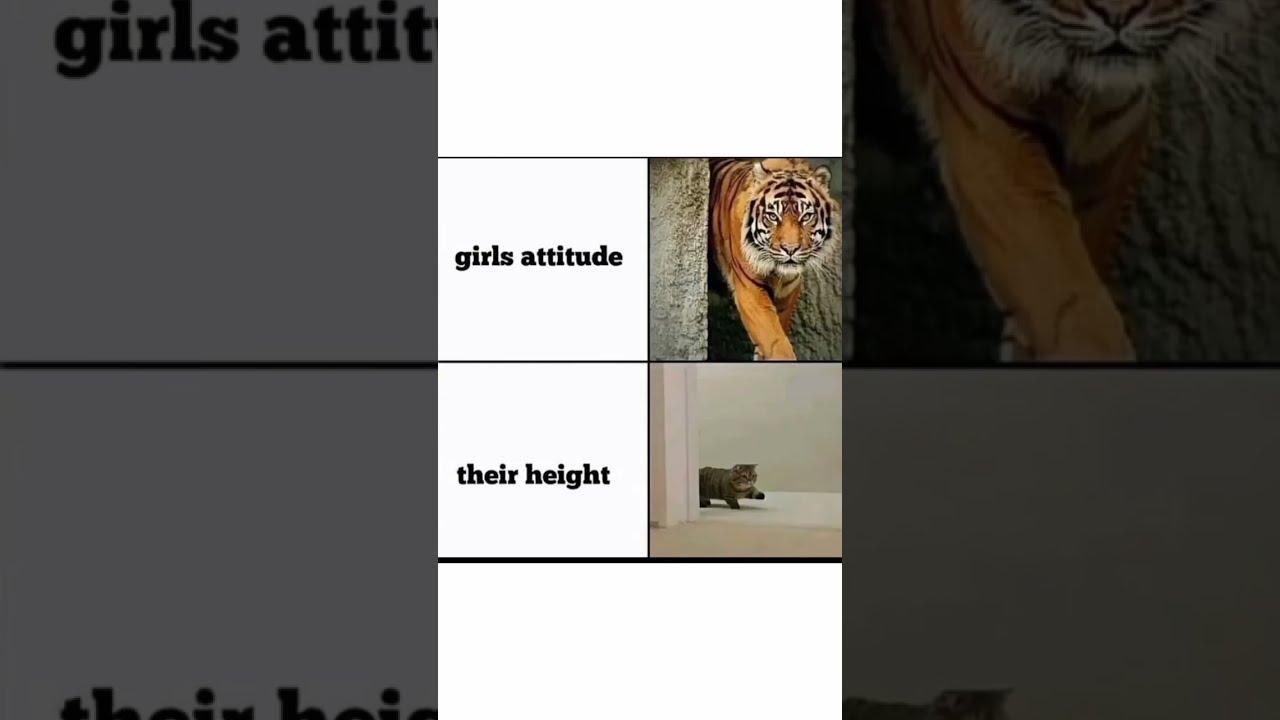The image is a meme with two panels, each with a white background, divided by a vertical line. The top left corner of the image features the text "girls' attitude" in bold, black, lowercase letters, next to a photo of a fierce, orange tiger with black stripes, partially emerging from a cave or a cement wall. The tiger, with a mix of white and black accents on its face, is set in an outdoor environment, possibly its natural habitat or a zoo. Below this, another white box with the text "their height" in the same bold black font is seen, next to an image of a small, stubby-legged kitten that resembles a gray tabby cat, walking out of a doorway. Surrounding the central meme are dark rectangular areas, adding a zoomed-in effect to the main image, creating a high-contrast and visually striking presentation befitting the humor of the meme.